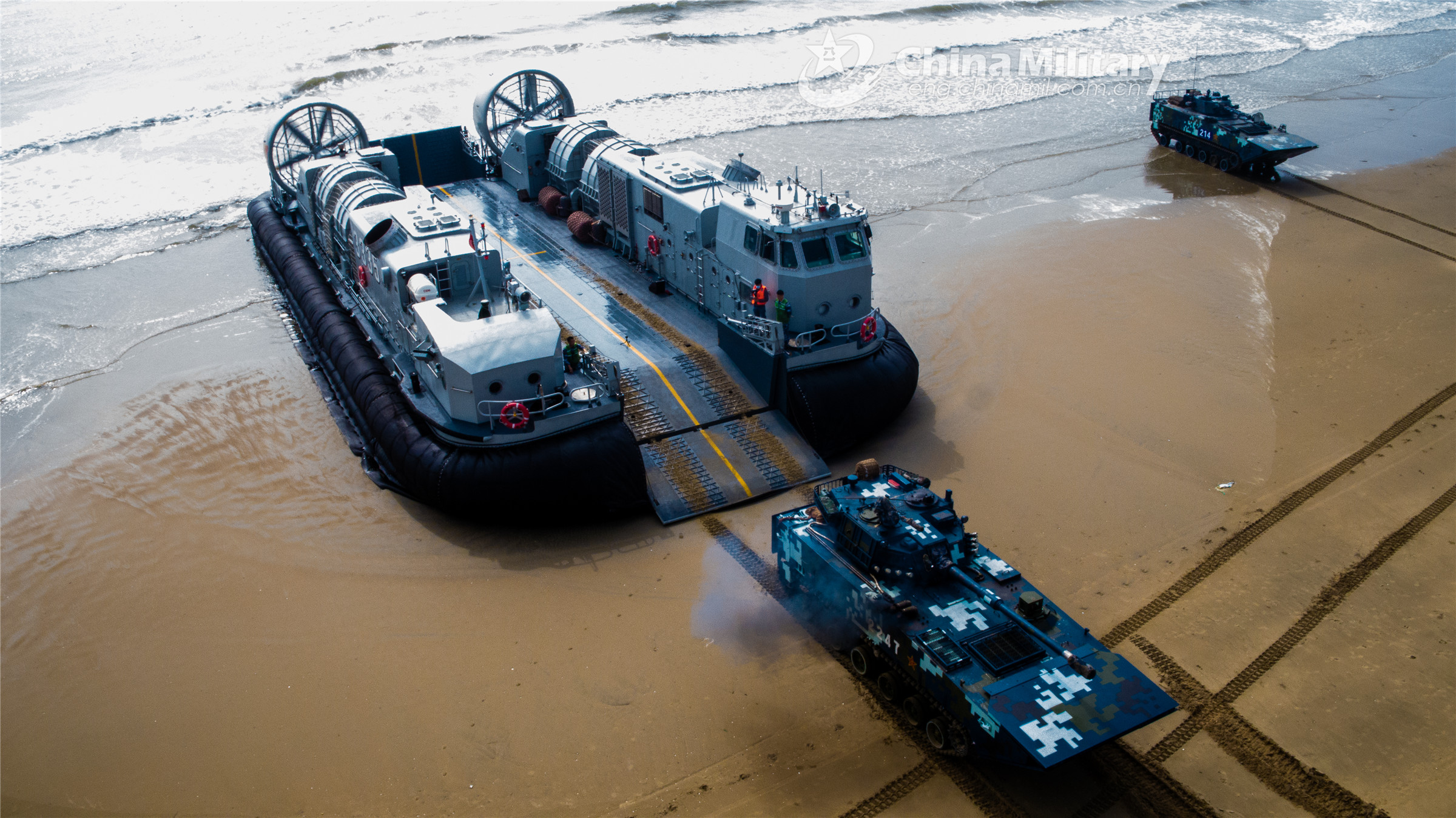The image depicts a Chinese military hovercraft, resembling the U.S. ELCAC landing craft air cushion system, beached on a sandy shore with the ocean in the background. The hovercraft, grayish and wet, has distinct yellow stripes on its ramp to guide vehicles. A dark-colored tank with a camo pattern is on the ramp, either moving off or onto the hovercraft. Tracks in the sand indicate prior movements of tanks. The hovercraft features large propellers or fans at the back. Another similar vehicle is visible a few feet away from the ramp, and on the right-hand side, there's another tank or vehicle appearing to back into the ocean. The scene is set under sunny conditions with the watermark "China Military" in the far right corner. People are seen standing around the vehicles, indicating possible human operation or supervision.